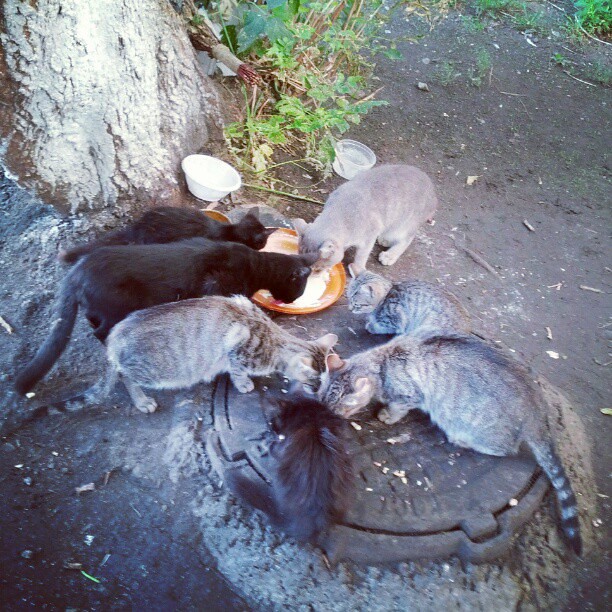The image is a slightly low-resolution photograph taken from above, showing a group of seven cats gathered outside. The scene is set around a manhole cover and a tree stump in an area with sparse greenery and mostly dirt ground. In particular, three cats—two black and one gray—are drinking from an orange bowl, likely containing milk, positioned adjacent to the manhole cover. Nearby, a small gray-striped kitten rests quietly. Close to the tree trunk, there is an overturned white ceramic bowl and a clear plastic bowl with water. On the manhole cover itself, four additional cats—two light gray with black stripes and spots, one primarily black, and another black cat—are gathered, seemingly eating food scraps. These cats appear to be a mix of adults and kittens, and their colors range from black to different shades of gray and brown. The overall impression is that these might be stray or wild cats that someone has kindly left food and water for.